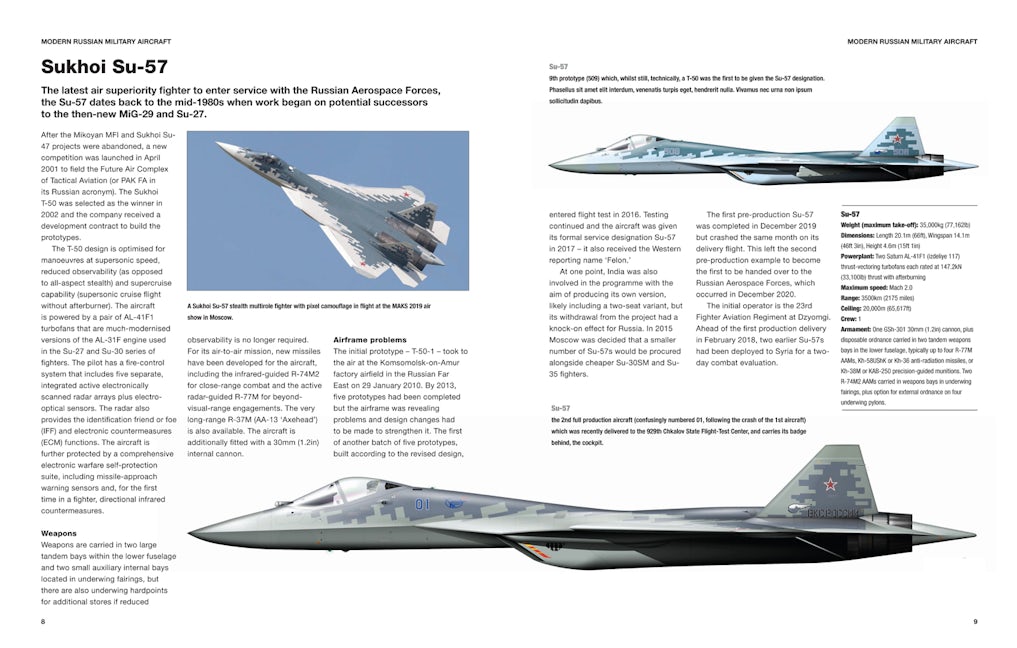The image depicts a leaflet about the Sukhoi Su-57, the latest air superiority fighter entering service with the Russian Aerospace Forces. The background of the leaflet is white, resembling a scanned piece of paper or a magazine spread, consisting of two pages with three columns each. On the upper left side, in bold black text, it states "Modern Russian Military Aircraft" followed by "Sukhoi SU-57." 

The primary image features a sleek, gray fighter jet with urban camouflage design, flying through a blue sky. The airplane showcases distinctive details like a red star on its tail, with additional white and blue segments on the tail fins. Below the main picture, there's a smaller image showing the jet from a slightly different angle, heading towards the left and displaying a reflection on its white windshield. 

Text accompanying the images describes the Sukhoi Su-57's specifications, including its weight, dimensions, power plant, maximum speed, range, ceiling, and crew capacity. There's also historical context provided, noting that the SU-57 project's origins date back to the mid-1980s as a successor to the MiG-29 and SU-27. The text is mostly black and small, making it difficult to read at a glance but offering detailed technical and historical information about this advanced Russian military aircraft.